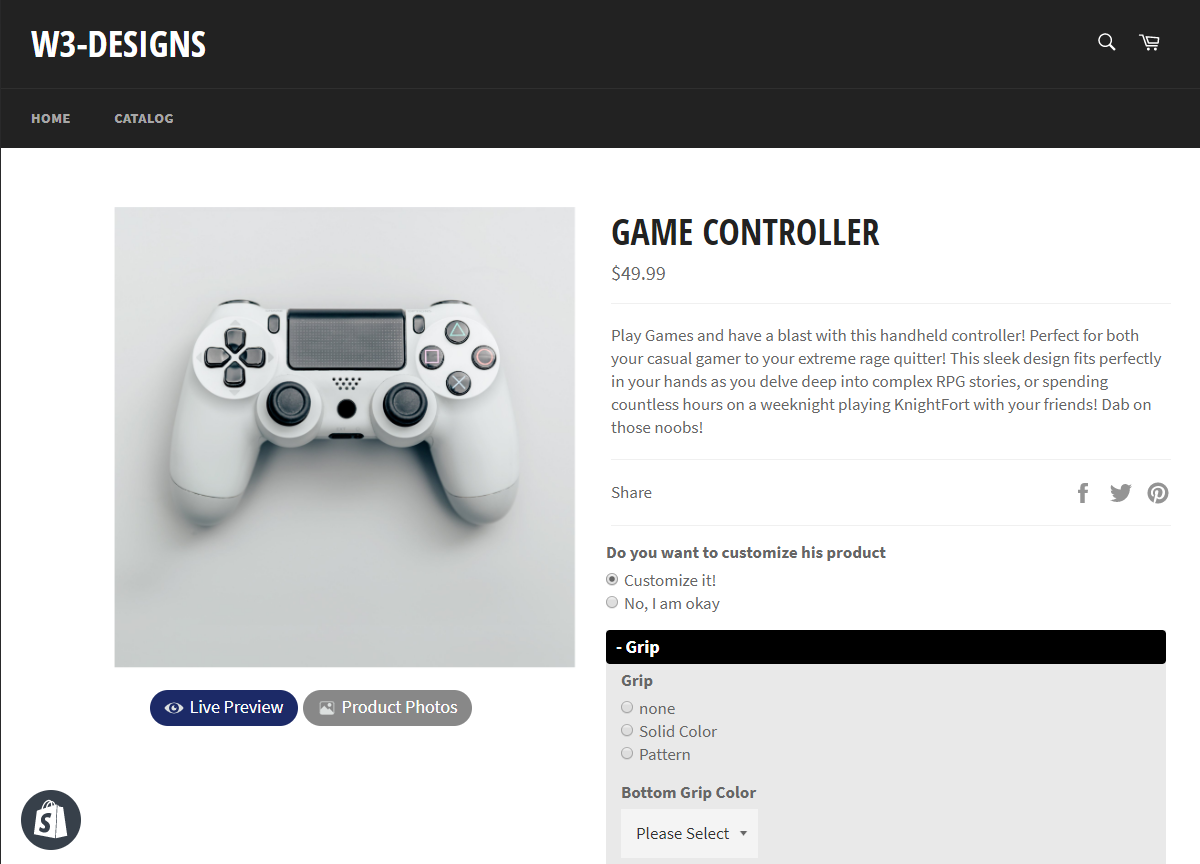This image is a screenshot from the website w3-Designs, showcasing a game controller available for purchase. At the top of the image, a black header bar displays the website name "w3-Designs" in white text, with navigation links to "Home" and "Catalog" underneath.

On the left side of the image, there is a grey box containing a picture of the game controller. Adjacent to the image, the text “Game Controller” appears in black, with a price of $49.99 listed below. 

A detailed description follows, highlighting the controller's appeal: “Play games and have a blast with this handheld controller. Perfect for both your casual gamer and extreme rage quitter. The sleek design fits perfectly in your hands as you delve deep into complex RPG stories or spend countless hours on weeknight gaming sessions, like playing Nightfort with friends. Dab on those noobs.”

Beneath the description, there are sharing options featuring icons for Facebook, Twitter, and Pinterest. 

The next section asks if you want to customize the product, though "this" is mistakenly spelled as "his." Below, there is an invitation to “customize it” and then a button labeled “I'm okay.”

Further down, another black-bar-topped, gray rectangular box titled “Grip” offers customization options. It lists three choices with checkable circles: “None,” “Solid Color,” and “Pattern.” Following these options, there’s a section labeled “Bottom Grip Color” with a “Please Select” button for additional customization.